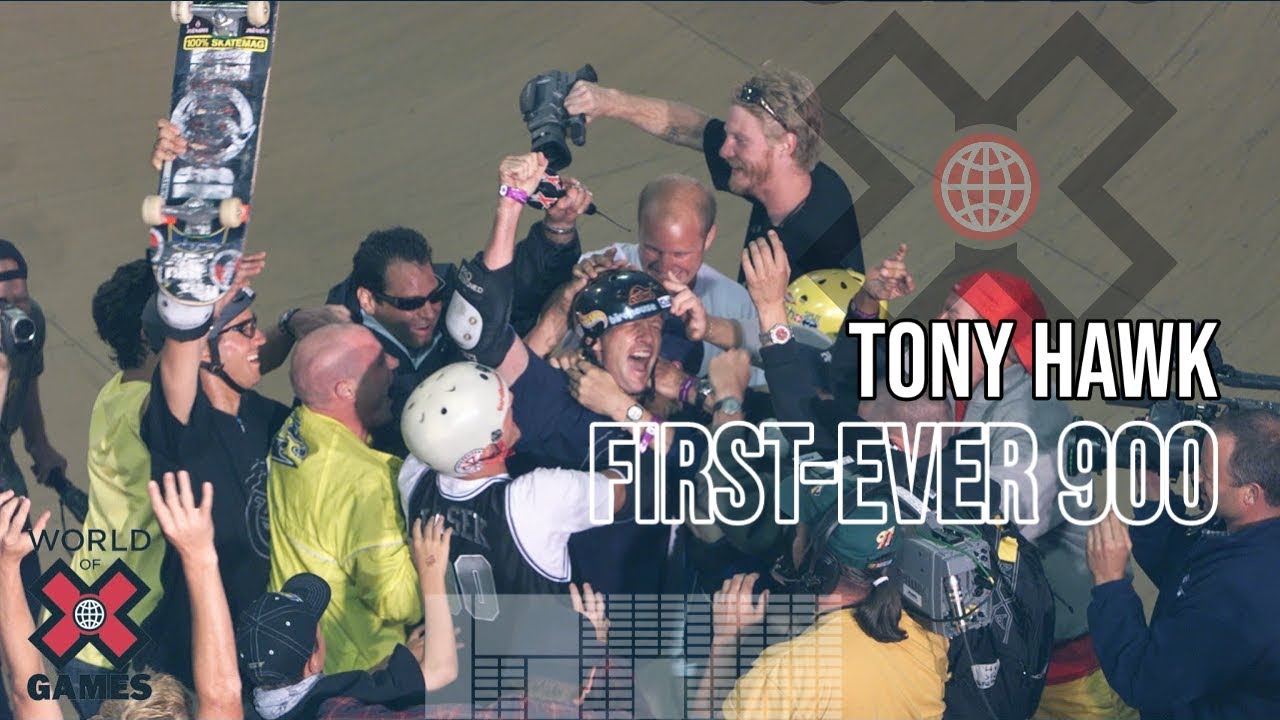This image captures the electrifying moment of Tony Hawk's historic achievement, landing his first-ever 900 at the X Games. At the center of the photo, Tony Hawk is beaming with joy, his mouth wide open in a smile, and his right arm triumphantly raised. Donning a helmet, his face is clearly visible, showing pure elation. A shoulder pad is discernible on his right elbow. Surrounding him is a jubilant crowd, including a skateboarder to the left hoisting a skateboard in celebration and a person above Tony with a hand on his helmet, likely pouring beer in celebratory fashion. The scene is bustling with activity as microphones and cameras are thrust toward Tony, capturing every moment of this landmark event. Overhead, a cameraman is positioned to record the entire scene. The image is branded with text noting "Tony Hawk first ever 900" and the bottom left corner features the "World of X Games" logo inside a red 'X.' Additional visual elements include a graph-like structure visible at the bottom, adding to the dynamics of the celebratory environment. This photograph vividly encapsulates the euphoric atmosphere surrounding Tony Hawk's monumental skateboarding milestone.